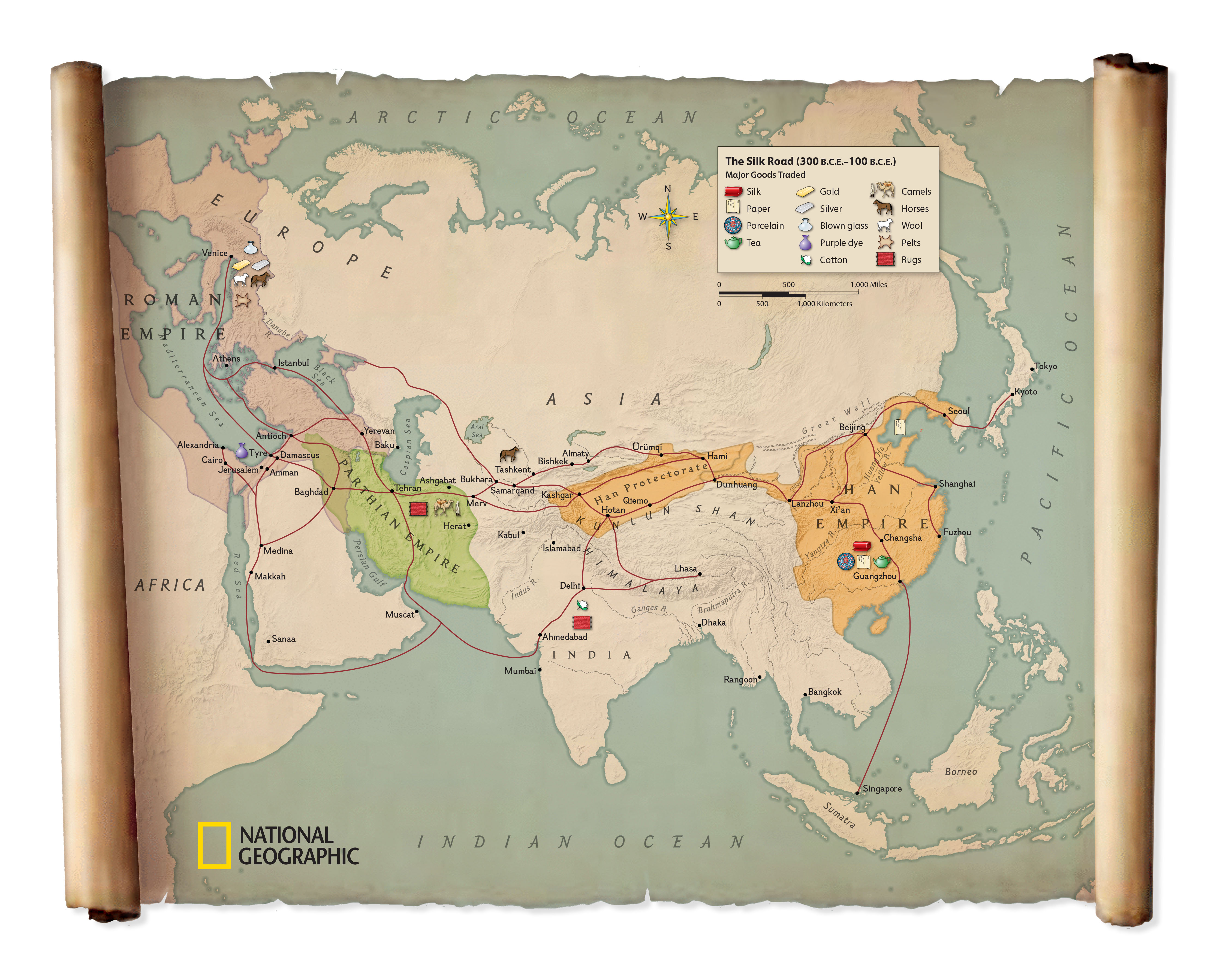The image is a computer-generated map centered on Asia, showcasing the ancient Silk Road routes from 300 BCE to 100 BCE. The map, by National Geographic, features a yellow square logo in the bottom left corner and has the appearance of an old, yellowed scroll with frayed top and bottom edges and rolled-up sides. The map details the Silk Road's historical trade routes marked in red, illustrating the vast network spanning Asia, Europe, and the eastern portion of Africa. In the top-right corner, there is a legend box indicating various trade goods through symbolic representations—red for silk, white for paper, blue for porcelain, a green teapot for tea, gold bars for gold, silver bars for silver, and a glass jar for blown glass. Additionally, the map includes depictions of oceans—the Arctic Ocean at the north, the Pacific Ocean to the east, and the Indian Ocean to the south—with the Roman Empire outlined to the west. The intricate legend also highlights trade elements like camels, horses, wool, pets, rugs, purple dye, cotton, and more, effectively mapping out the origins and trade routes of these goods across the regions.